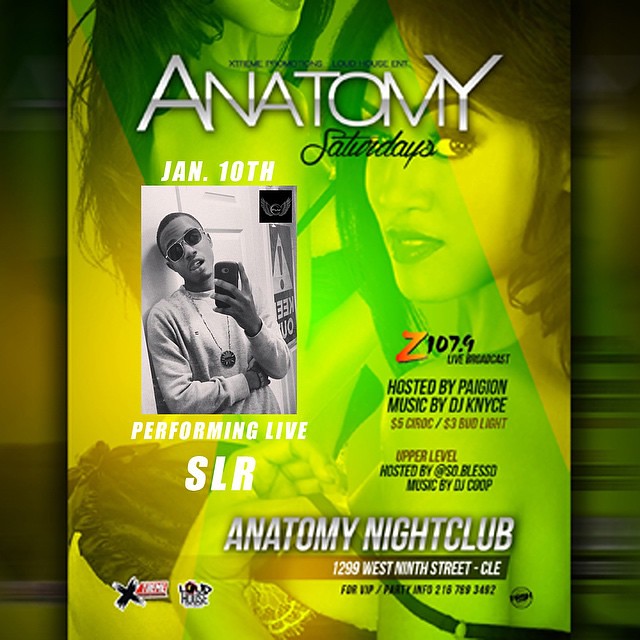The image appears to be a promotional flyer for a nightclub event titled "Anatomy Saturdays." The word "Anatomy" is prominently displayed at the top in white with a gray gradient at the bottom of the letters, while "Saturdays" is written in a stylish black script beneath it. 

In the background, there are photos of a few attractive women adding to the overall aesthetic. Central to the flyer is a photo of a gentleman wearing glasses, holding a cell phone, and adorned with a pendant around his neck. He is dressed in a long-sleeve shirt.

Above this central image, the date "January 10th" is written in white lettering. Below, it states "Performing Live SLR." To the right of the gentleman's photo, there is a prominent red "Z" symbol, indicating the involvement of Z107.9. It has the text "Z107.9 Live Broadcast hosted by Pagan Music" and mentions "DJ Nice."

Further down, the flyer lists various pricing details, although parts of it are not fully visible. At the bottom, it clearly indicates the venue information: "Anatomy Nightclub," located at "1299 West 9th Street, Cleveland."